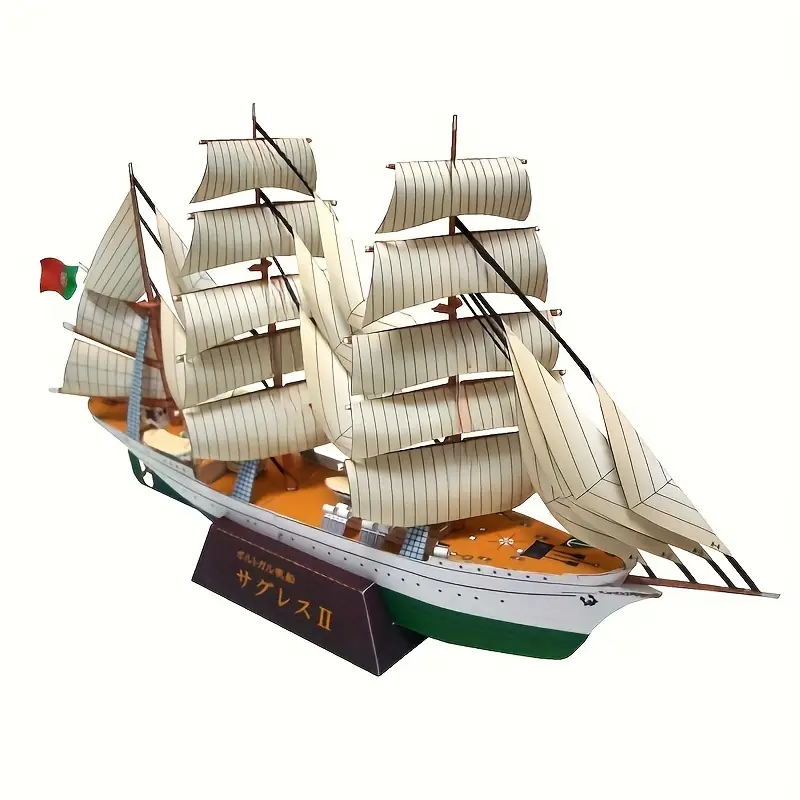This photograph showcases a detailed model of a grand tall ship, a miniature representation of what would be an imposing and impressive sailboat. The ship features three prominent masts, with the two main masts each bearing five rectangular vertical sails. At the rear, a smaller mast displays three vertical sails, adding to the ship’s complex rigging system. Another mast extends from the bow, with additional sails stretched between straps leading to the first main mast. Notably, there is a large, triangular rear sail as well. Adorning the vessel, which rests on a brown stand inscribed with gold Asian characters, is a Portuguese flag. The ship's hull boasts a distinct green keel below the waterline, and the section just above is pure white, marked with small black horizontal dots. The deck is a vibrant orange, and additional smaller characters are painted across it, possibly indicating a compass rose. Labels on the sails are present but too small to decipher. The intricacies and cultural elements make this model a remarkable and captivating representation of a traditional tall ship.